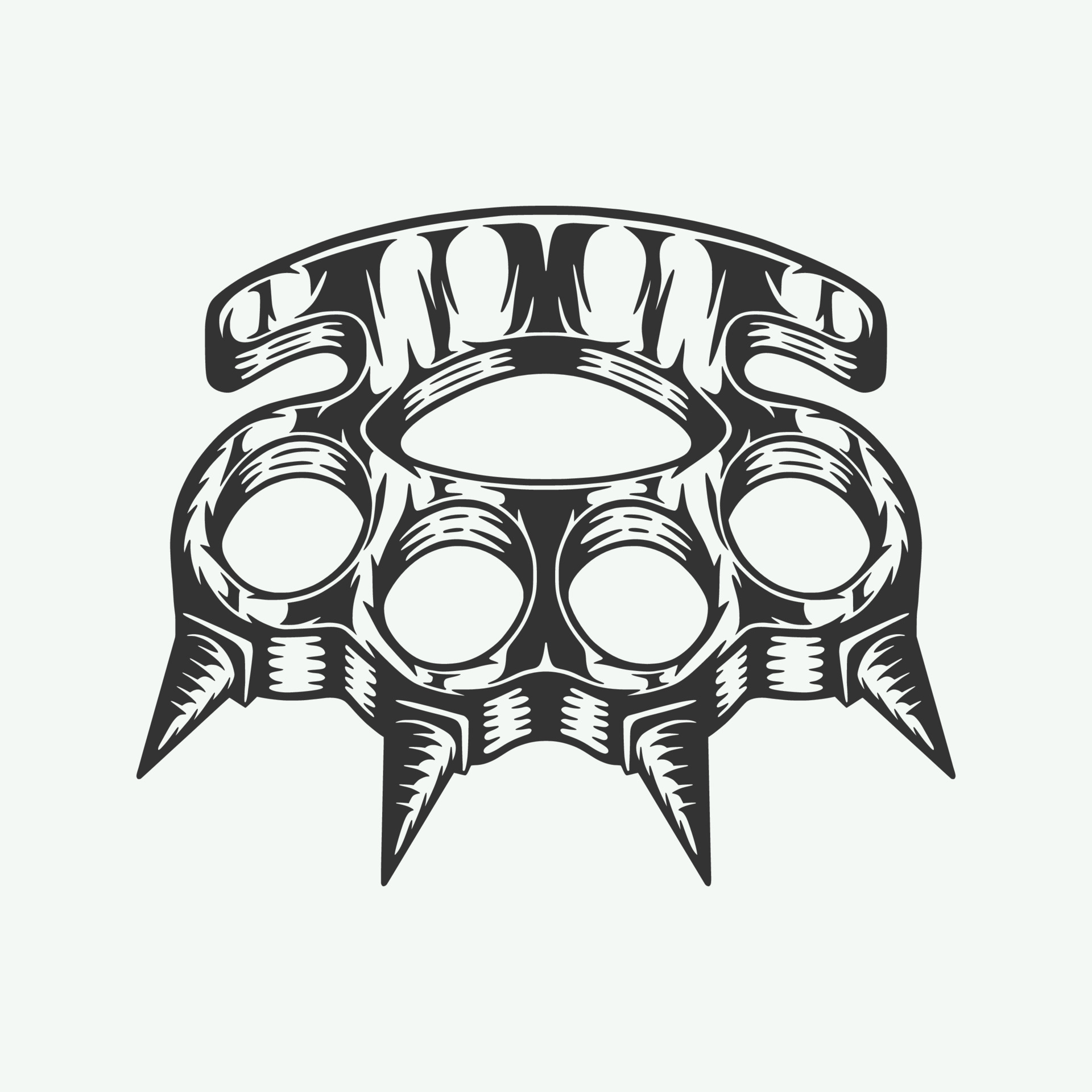The image depicts a detailed, black and white drawing of brass knuckles on a plain off-white background. The brass knuckles are illustrated with heavy, dark black lines, showcasing four finger holes and an additional larger hole that would fit into the palm when gripped. Above each finger hole is a sharp spike, each spike resembling a traffic cone with a square base, arranged in a triangular formation. The brass knuckles also feature an intricate, symmetrical pattern of wisps and designs, some resembling fences and others more abstract shapes, which add to the three-dimensional appearance of the print. The overall shape curves slightly upward at the top, enhancing the menacing look of the drawn brass knuckles.